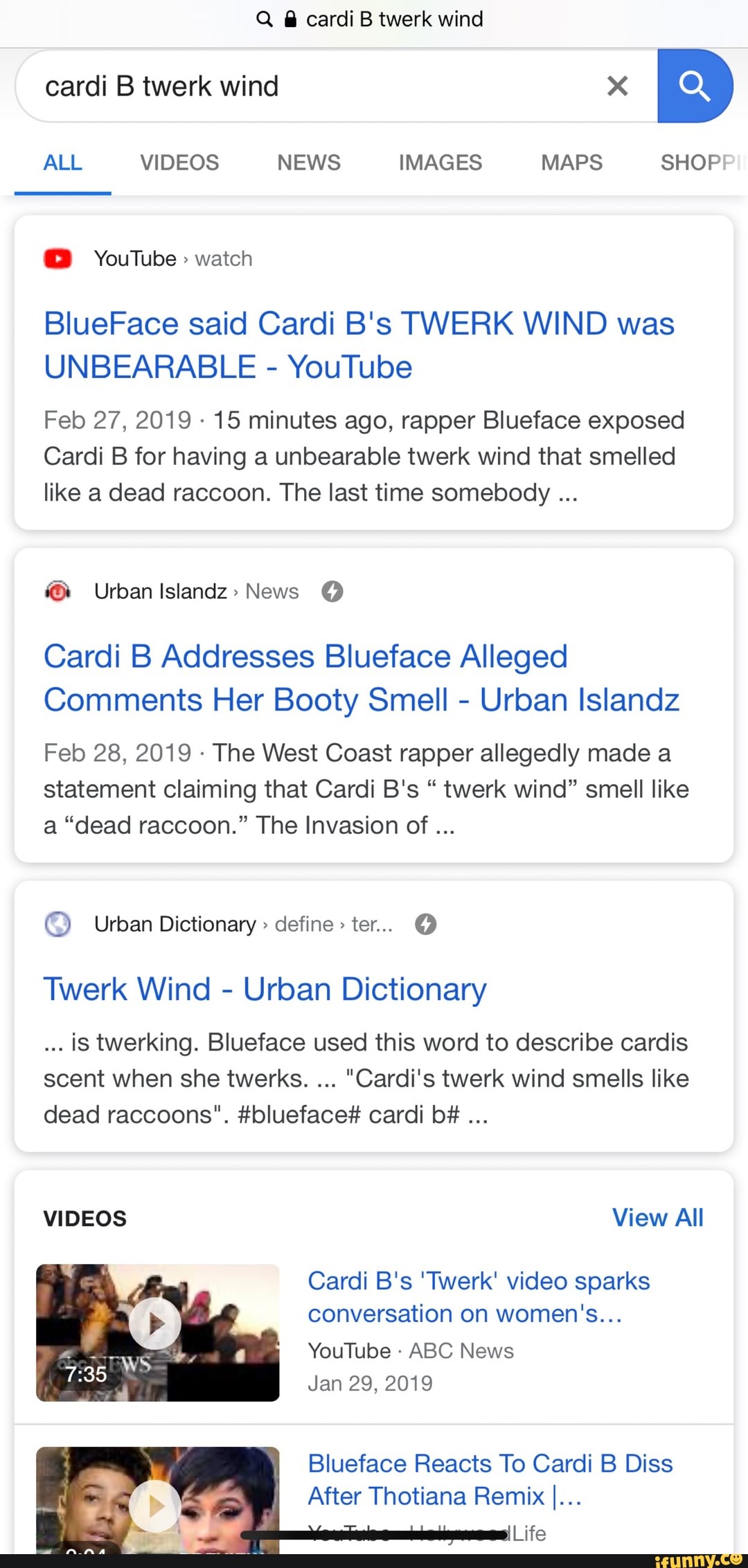The image displays a Google search results page for the query "Cardi B twerk win." At the top, there is a Google search bar with a magnifying glass icon and a lock icon, indicating a secure search. The search term "Cardi B twerk win" is visible inside the search bar, accompanied by an "X" button and another magnifying glass button.

Below the search bar, several category tabs are outlined, including "All," "Video," "News," "Images," "Maps," and "Shopping."

The first result listed is from YouTube, displaying a video titled "Blueface said Cardi B's twerk win was unbearable," uploaded on February 27, 2019. The description mentions that rapper Blueface criticized Cardi B for having an unbearable twerk win, likening its smell to that of a dead raccoon.

The second result is from Urban Islandz News, with an article titled "Cardi B addresses Blueface's alleged comment about her booty smell," dated February 19, 2019. The snippet explains that West Coast rapper Blueface allegedly claimed that Cardi B's twerk win smelled like a dead raccoon.

The third result is from Urban Dictionary, providing a definition for the term "twerk win."